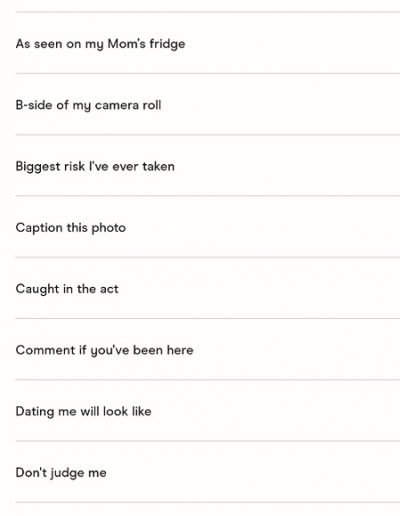The image features a vertically arranged list of eight captions, each separated by thin, light gray horizontal lines. The background is white, making the text stand out clearly. From top to bottom, the captions read as follows:

1. As seen on my mom's fridge
2. Beside my camera roll
3. Biggest risk I've ever taken
4. Caption this photo
5. Caught in the act
6. Comment if you've been here
7. Dating me will look like
8. Don't judge me

Each segment is neatly typed, creating a clean and organized appearance. The light gray lines between each caption provide subtle separation without overwhelming the overall simplicity of the design.